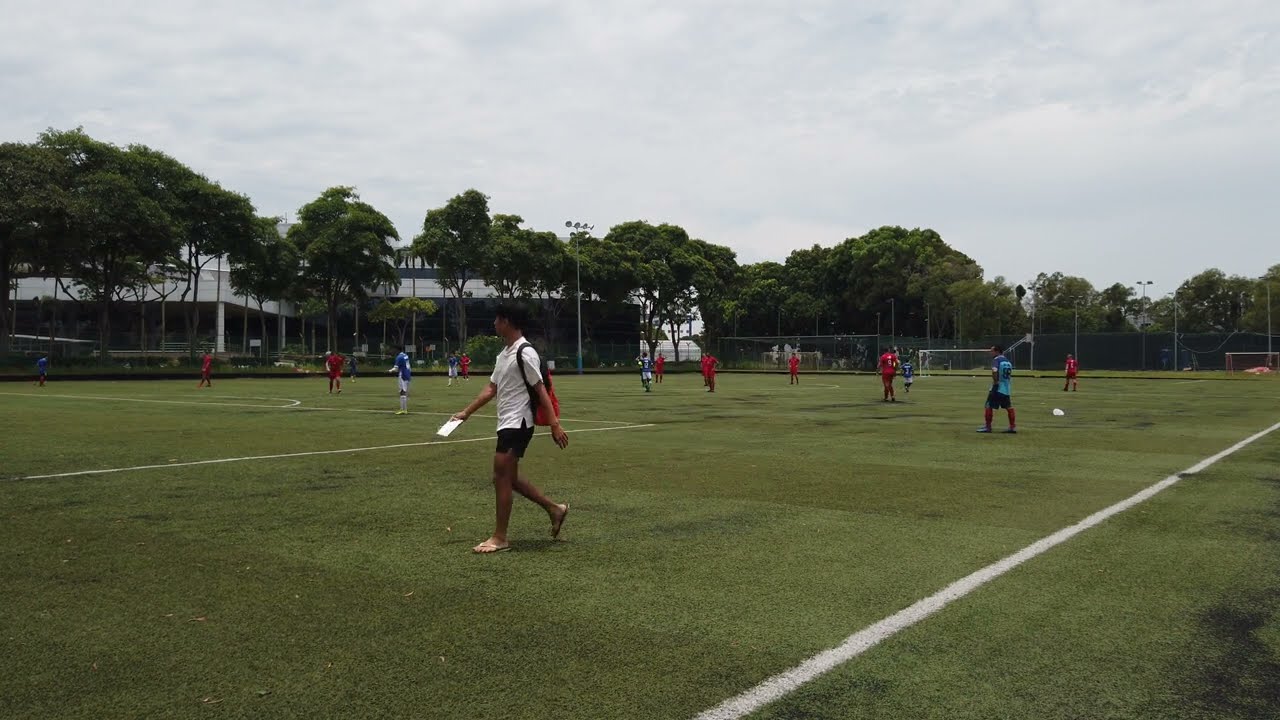The photograph captures a well-manicured yet somewhat worn soccer field, with evenly cut green grass marred by patches of blackened, weathered spots. White lines crisply delineate the field's sections, guiding the action of multiple players engaged in what appears to be either a match or practice. These players are split into two teams, one donning red jerseys paired with red pants, and the other in blue jerseys complemented by white shorts. 

In the center of the field, a man distinct from the players casually strolls in flip-flops, wearing a white shirt and a backpack, suggesting he is either a coach or a spectator stepping onto the field. The far end of the field features a white soccer goal, framed elegantly by a fence line that separates the playing area from its periphery.

Beyond the fence, a row of lush, green deciduous trees provides a natural boundary, their leaves adding a touch of vibrancy to the scene. Behind these trees, several buildings punctuate the landscape, while above them, the sky stretches out in a vivid blue palette adorned with scattered white clouds, completing the picturesque sporting environment.